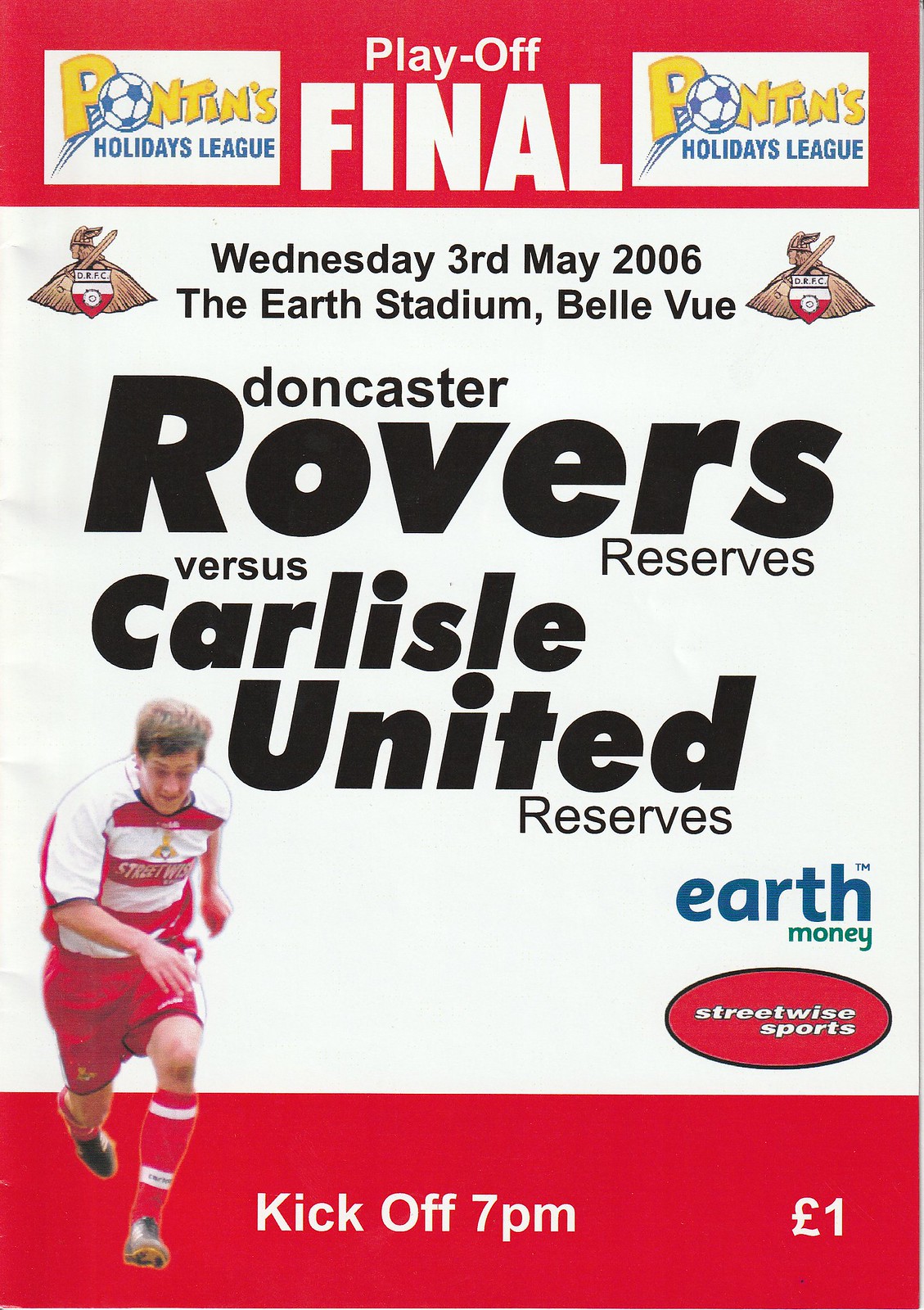The image is a digital poster for a playoff final in the Pontins Holidays League. At the top, there's a red banner with white text that reads "PLAY-OFF FINAL." Flanking this title on the left and right are small white boxes with yellow text stating "PONTINS," where the 'O' is stylized as a soccer ball. Below that, in blue text, it says "HOLIDAYS LEAGUE." The main part of the poster features a white background with black text detailing the event: "WEDNESDAY 3RD MAY 2006," "THE EARTH STADIUM, BELLEVUE," and "DONCASTER." Prominently in large black capital letters, it says "ROVERS," followed by "RESERVES" in smaller font. To the left of this, it says "VERSUS," and below that, also in black font, it says "CARLISLE UNITED RESERVES." At the bottom left of the poster, there's an image of a football player in a red and white striped jersey, red shorts, and red socks. Underneath this image, in a red box with white text, it says "KICK-OFF 7 PM" and mentions the entry fee is "£1."